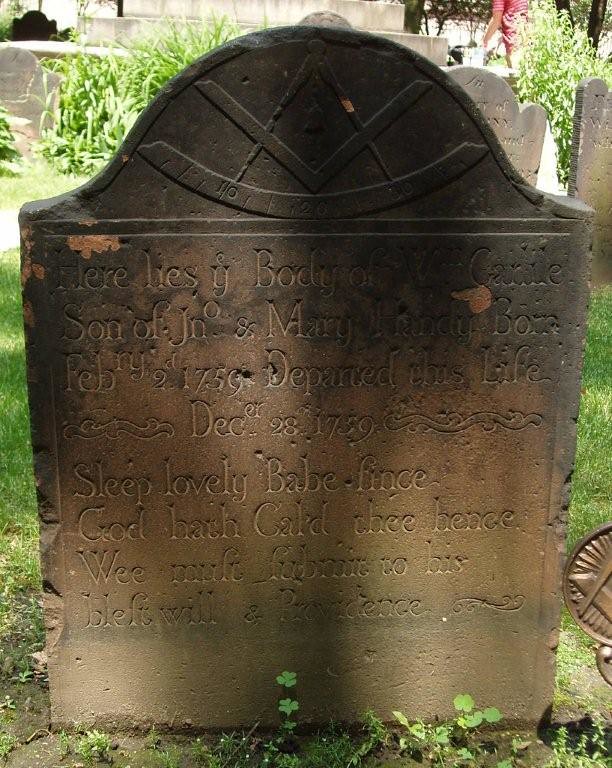The photograph showcases an aged and weathered headstone from the 1700s, exhibiting a brownish hue suggestive of a possible copper material. The gravestone is intricately designed with curvy, engraved text that reads, "Here lies the body of Carney, son of John and Mary, born on February 2nd, 1759, departed this life on December 28, 1759. Sleep lovely babe, for God hath called thee hence, we move to his will and providence." At the top of the headstone, a distinctive symbol featuring an angle and an upside-down angle with a little banner underneath is noticeable, though somewhat degraded over time. The backdrop features verdant vegetation and similar headstones, contributing to an atmosphere of historical solemnity. Near the base of the photograph, grass and clovers add an element of natural serenity to the scene.